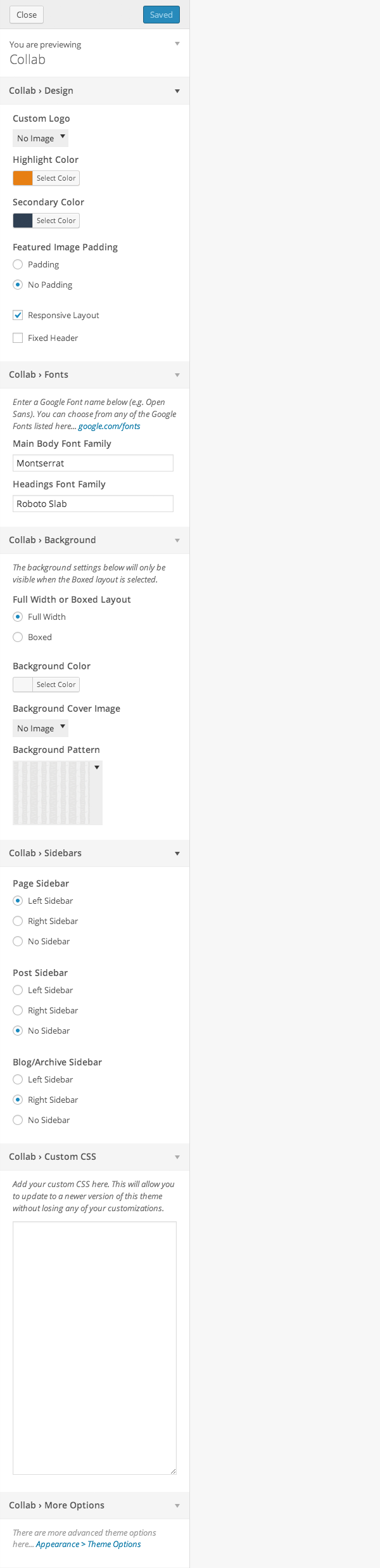**Caption:**

The image, oriented vertically, appears to be a screenshot from a computer or smart device, displaying a customizable interface. At the top of the screen, a gray bar features options for closing the screen on the left and saving changes in a teal blue on the right. Below the bar, on a white background, a message reads, "You are previewing collab."

Following this message, a set of customization options is displayed within a gray box labeled "collab design." Users can navigate through various settings:

1. **Custom Logo:** No image selected, with an option to upload.
2. **Highlight Color:** Currently set to orange, with an option to change.
3. **Secondary Color:** Currently set to black, with an option to change.
4. **Featured Image Padding:** Options for padding (currently set to no padding).
5. **Responsive Layout:** Checked.
6. **Fixed Header:** Not checked.

Continuing, the "collab fonts" section allows users to:
- Enter a Google font name, using the example "Open Sans."
- Choose from any Google fonts provided via a web address link.
- Set the main body font family to Montserrat.
- Set the headings font family to Roboto Slab.

The "collab background" section specifies that the background setting will only be visible when the box layout is selected. Users can pick a background color, cover image, or background pattern. Additionally, the same customization options are available for sidebars, including post sidebar, blog archive sidebar, collab custom CSS, and collab more options for advanced theme customization.

For further customization, users can click on "appearance" or "theme options," both hyperlink text in blue.